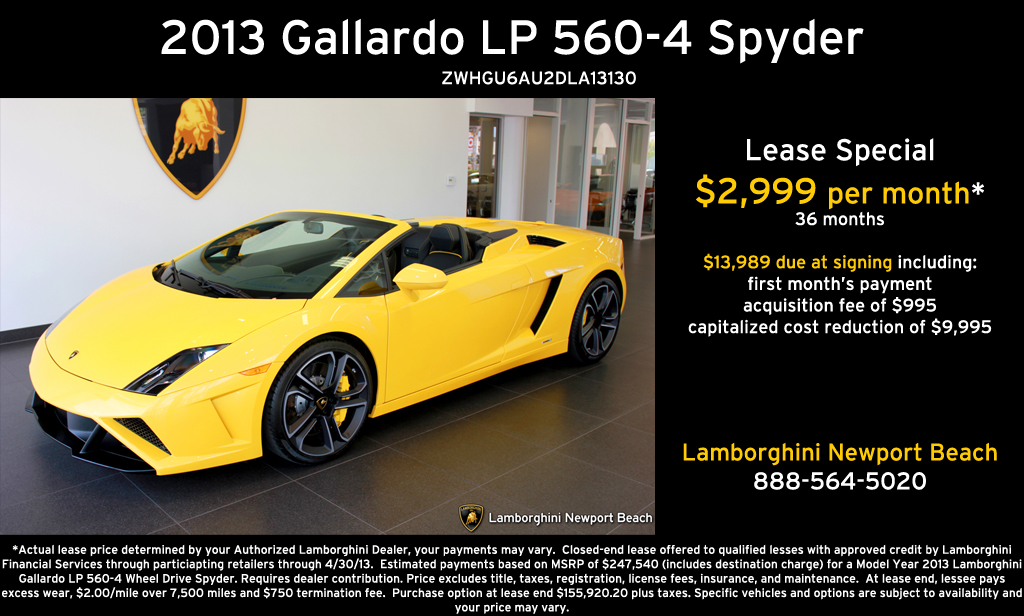This image is an internet advertisement for leasing a 2013 Lamborghini Gallardo LP 560-4 Spyder, prominently featuring a yellow convertible model on the left side against a black background. The title, "2013 Gallardo LP 560-4 Spyder," is written in bold white text at the top. On the right side, the lease special is detailed: $2,999 per month for 36 months, with $13,989 due at signing. This amount includes the first month's payment, an acquisition fee of $995, and a capitalized cost reduction of $9,995. Below these details, the ad specifies "Lamborghini Newport Beach" in yellow text, followed by a contact number, 888-564-5020, in white text. Additional disclaimers and terms about the lease are written in fine print at the bottom of the image.